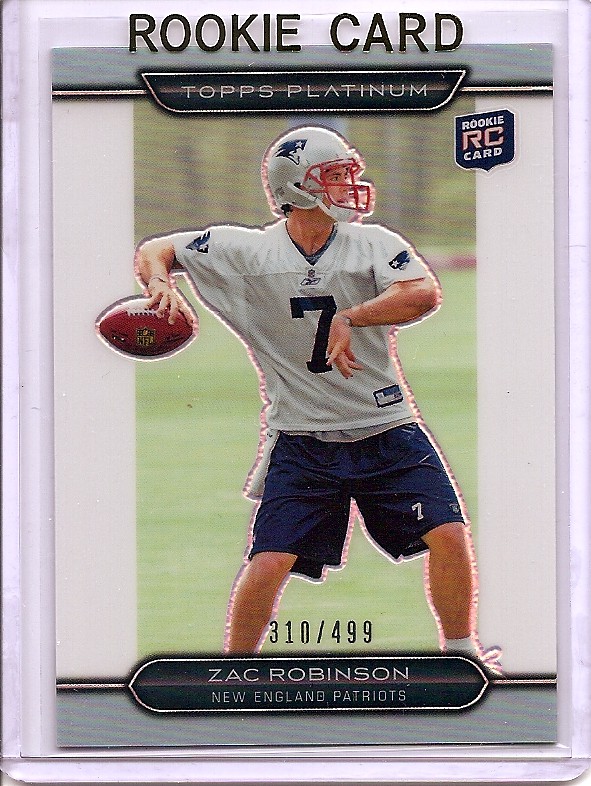This image showcases a rookie football card of Zach Robinson, specifically a Topps Platinum edition. The card itself is housed within a clear plastic top loader for protection. At the top of the card, "ROOKIE CARD" is printed in uppercase black letters, followed by "Topps Platinum" in a distinctive, black trapezoidal framework. The card features an image of Zach Robinson, who is depicted in the midst of football drills, wearing a gray Patriots helmet and a white Reebok jersey with the number 7. His dark blue shorts also display the number 7. Robinson is poised with a football grasped in his right hand, ready to throw, as his left hand is positioned to his side. The background reveals a grassy field, adding context to the camp setting. Below the image, the card is serially numbered as 310 out of 499, with the inscription "Zach Robinson" and "New England Patriots" at the bottom.